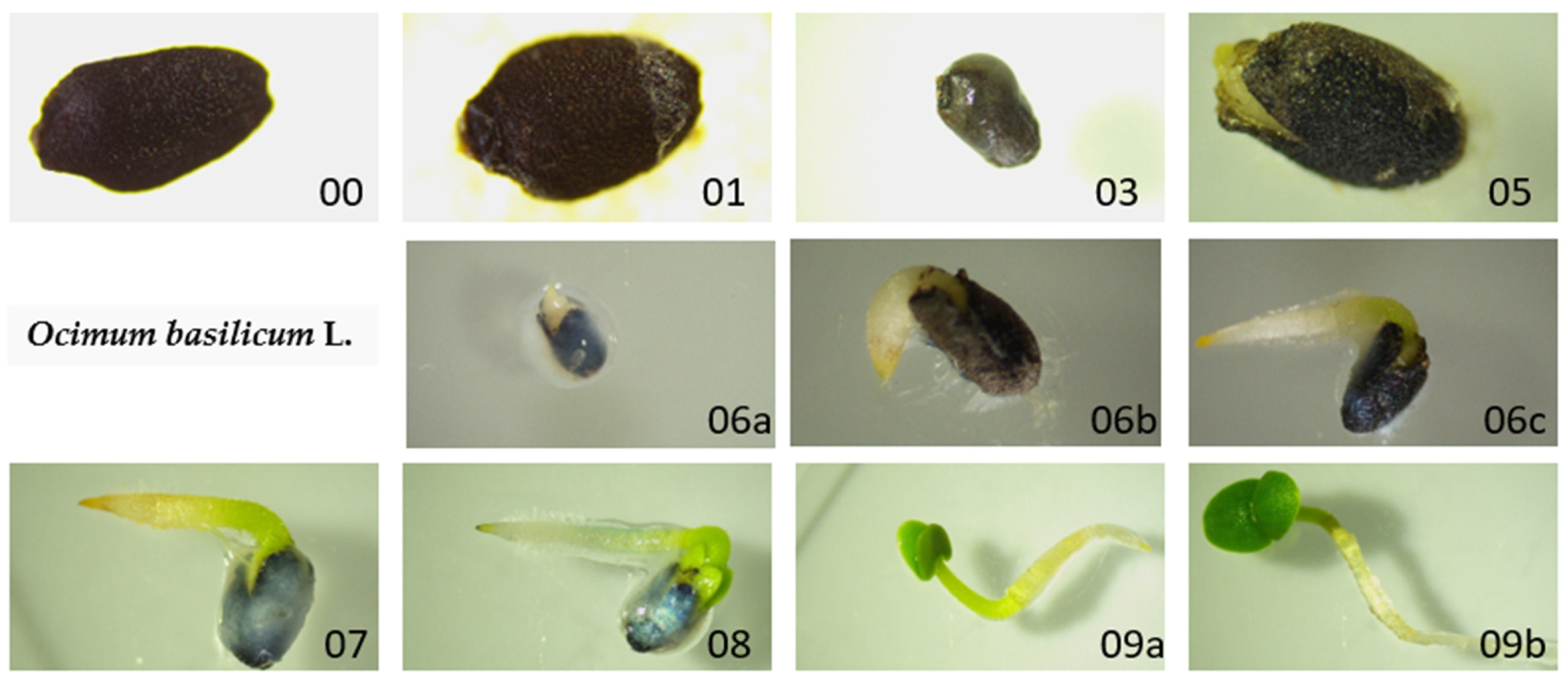This image is a detailed collage showcasing the various stages of basil plant growth, featuring 12 distinct images. Each image is meticulously labeled on the bottom right corner with numbers from 00 to 09, including additional labels such as 6A, 6B, 6C, 9A, and 9B. The top-left image displays a black oval shape labeled 00. Moving to the right, the subsequent images closely follow the progression of basil, from soil and black oval shapes to a yellow glowing pattern at the border (01) and other intermediate stages. The series traces the development from seed, represented as small black ovals, through different phases until small green sprouts emerge. The image array contains varied colors such as brown, black, gray, green, and blue, providing a vivid representation of basil (scientifically known as Ocimum basilicum L) sprouting. The final row showcases the basil with small green leaves, accentuating the culmination of the growth process.